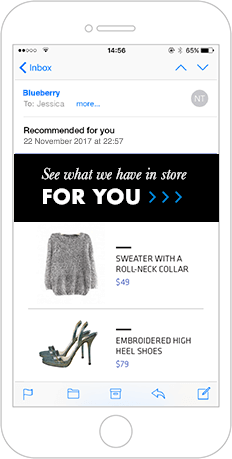The screenshot depicts a webpage with a clean, gray-bordered interface primarily showcasing black and white text with minimal color accents. At the top of the webpage, the text "Inbox" is displayed, indicating a personalized message or advertisement. Next to "Inbox," a timestamp reads "14 hours and 56 minutes," and to the right, there appears to be a bar indicating either the user's power level or rating. 

Prominently featured is a message that reads, "See what we have in store for you," suggesting a series of personalized product recommendations. The word "Blueberry," presumably the company name, is highlighted in blue, adding a touch of color to the otherwise monochromatic scheme. Below "Blueberry," the page is addressed to "Jessica."

Beneath the header, there is a detailed item description and timestamp, "November 22nd, 2017 at 22:57," and another instance of "See what we have in store for you." The main content features a product image of a sweater with a roll neck collar, accompanied by a description. Further down, another product is listed: embroidered high heel shoes. 

At the bottom of the page, there appear to be clickable options or buttons, though their specific functions are not clearly visible. Overall, the webpage provides a structured and user-specific shopping interface, with key elements in blue to emphasize the brand identity amid the largely grayscale design.